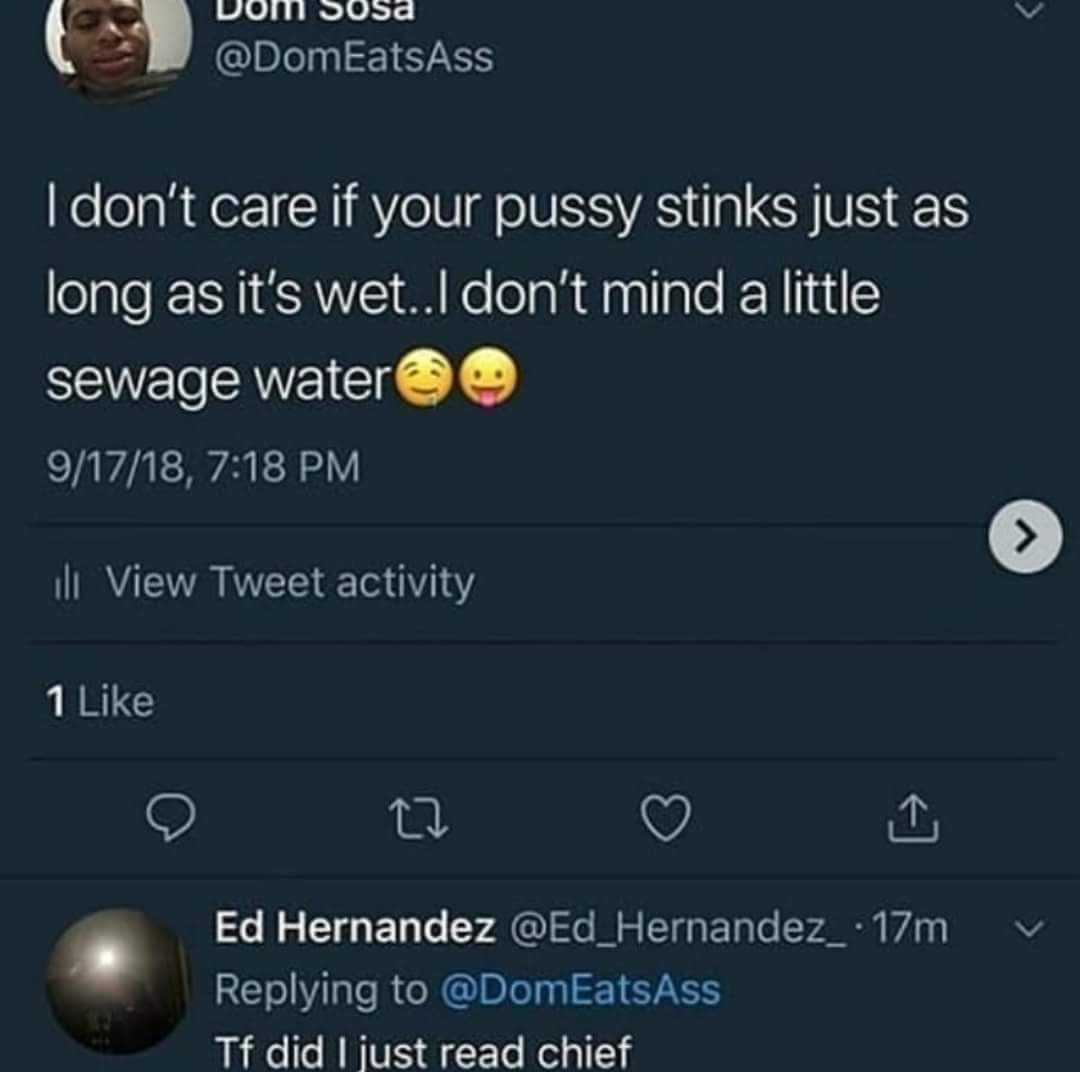This image is a detailed screenshot taken from the Twitter application, likely on a computer, showcasing a tweet by Dom Sosa, whose screen name is @DomEatsAss. The tweet, dated September 17, 2018, at 7:18 p.m., reads: "I don't care if your pussy stinks just as long as it's wet. I don't mind a little sewage water," and is accompanied by two explicit emojis (one drooling face and another with its tongue out). The background is predominantly dark blue, which is characteristic of the Twitter interface, and text elements appear in white. The screenshot reveals that the tweet received one like and features a comment by Ed Hernandez (@EdHernandez), who replied with: "TF did I just read, chief?" The entire image is dominated by this Twitter exchange, with no other significant objects or elements present.